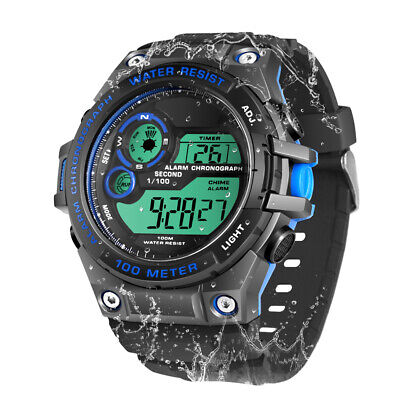This image is a detailed photograph of a sporty digital watch, seemingly suspended in a white void. The watch, primarily black with bright blue accents, appears to be made of durable rubber and plastic materials. Around the bezel, various functionalities are noted: in blue, it says "water resist" and "chronograph," and in white, it states "light," "ADJ," "100 meter," and "alarm chronograph."

The main display has a green backlight with black digits, showcasing measurements and reads "26" along with "second 100" in white, displaying a time of 9:28:27 seconds. A notable feature is the compass marking (NWES) at the top left of the display. Buttons around the bezel vary in color, featuring black and light blue, contributing to the watch's overall sporty aesthetic and usability.